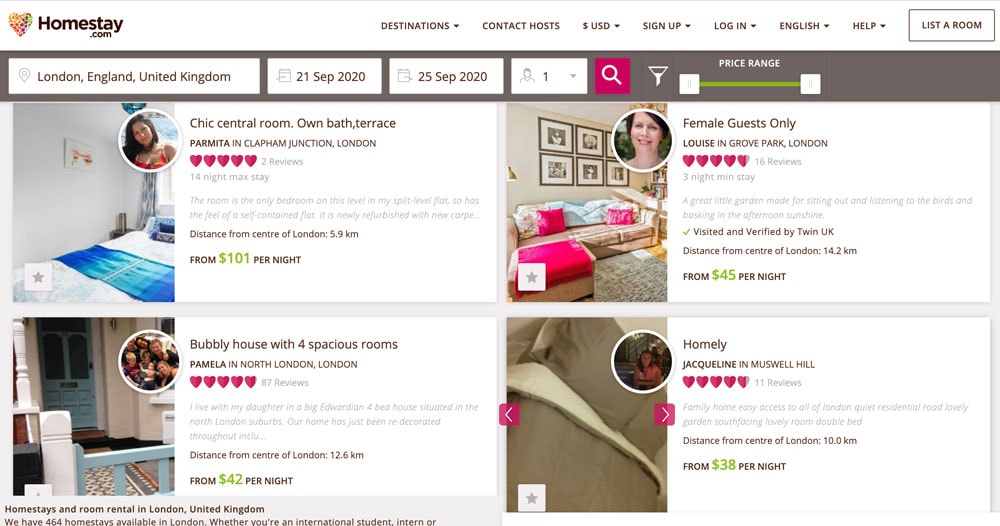Title: Accommodations on Homestay.com

Caption: The provided image is a screenshot from the website Homestay.com, showcasing various rental options and site functionalities. The top navigation bar features tabs labeled "Destinations," "Contact Host," "US Dollar," "Sign Up," "Login," and "English," along with buttons for "Help" and "List a Room." Two rental listings are prominently featured with detailed descriptions and pricing.

1. The first listing advertises a chic, central room in London, offering exclusive amenities such as a private bathroom and a terrace. This room is the sole bedroom on its level in a split-level flat, giving it the ambience of a self-contained apartment. The room has been recently refurbished with new carpeting and is available from $101 per night. The host’s profile picture shows a dark-haired woman in a bathing suit at the beach, appearing to be around 32 years old.

2. The second listing describes a lovely house with four spacious rooms, hosted by Pamela in North London. With 87 reviews, this rental is described as a large Edwardian house located in the North London suburbs. The property, which is newly redecorated, is available from $42 per night. Pamela lives with her daughter in this charming residence. 

In summary, the image captures a user interface replete with various booking options, key functionalities for visitors, and detailed host profiles and accommodation descriptions.